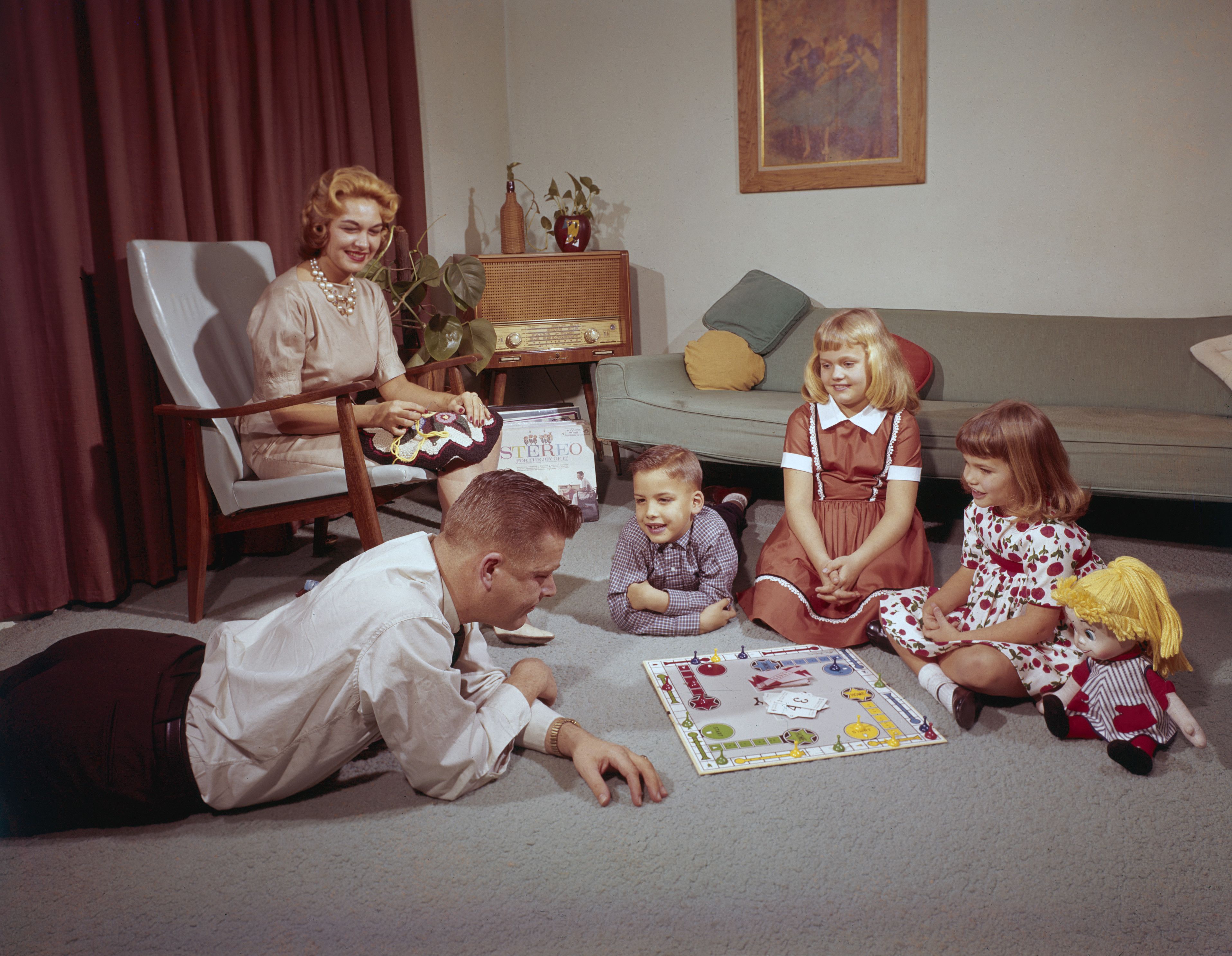The photograph vividly captures a nostalgic family scene in what looks like a 1950s living room. The room has white walls adorned with a gold-framed painting and a red curtain draping from the top left corner. The floor is covered in a gray carpet. Centrally, a man in a white shirt and dark pants lies on the floor, engaging intently with a board game, which might be the game of "Sorry," alongside three young children—two girls and one boy. The boy wears a gray shirt with dark pants, the first girl is dressed in a brown dress with a white collar, and the second girl sports a red and white printed dress. A blonde-haired doll is placed next to the children, adding to the playful ambiance.

Behind the family, a sofa with green upholstery is adorned with yellow, green, and white pillows. The setting is further enriched with a piece of vintage wooden stereo equipment, complemented by a plant in a brown vase. Seated gracefully on a wooden chair with white cushions, the mother, attired in a light tan dress with pearl accessories, is engrossed in embroidery, her blonde hair tied back as she smiles contentedly. The overall scene, filled with cheerful anticipation, highlights the family's shared moment of leisure, perfectly encapsulating the essence of mid-20th-century domestic life.